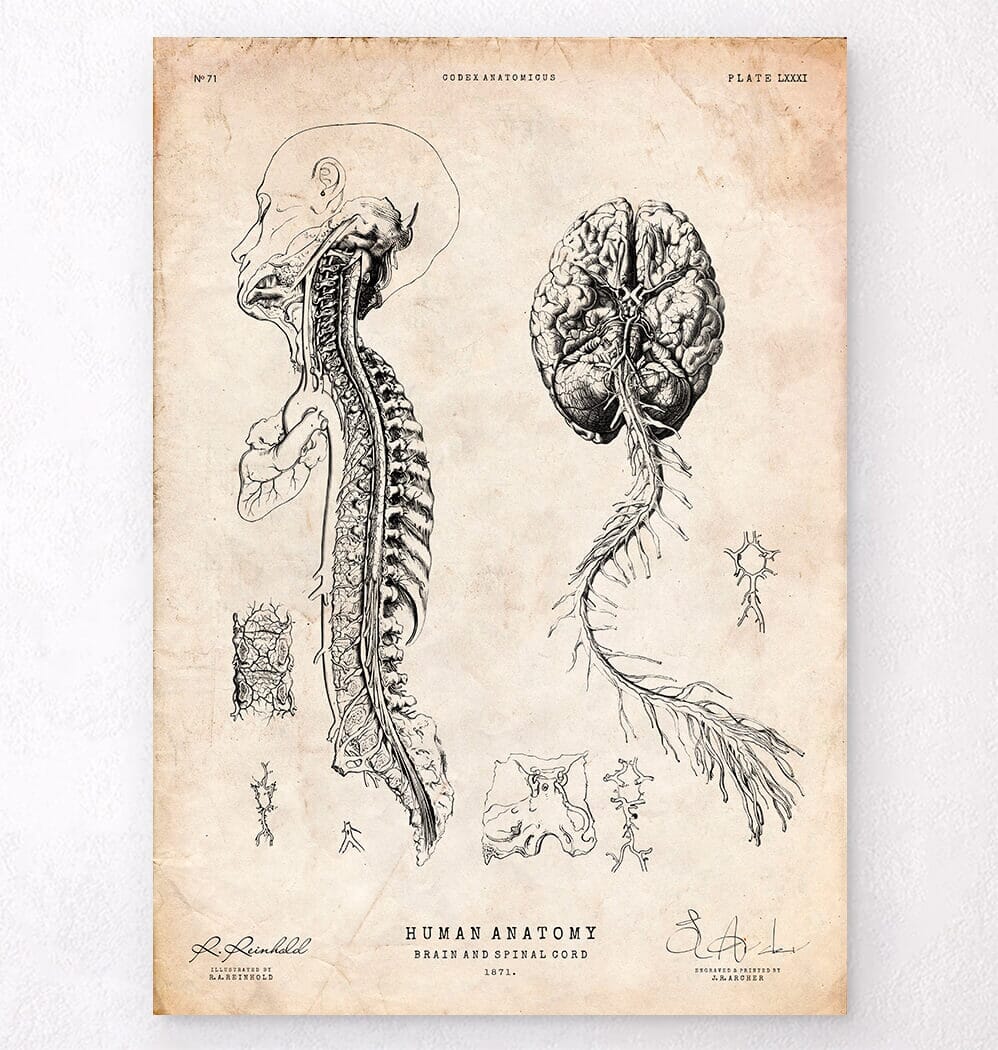The illustration is a vintage, black-and-white pencil drawing from an anatomy identification book, dating back to 1871. The background is an aged, cream-tone parchment that darkens toward the edges, enhancing its antique appearance. On the left-hand side, the drawing features a detailed profile of a human head, showing the skull and face turned to the left, with a comprehensive depiction of the spinal cord extending downward. The right-hand side showcases an intricate view of the brain from the underside, detailing the lobes, sulci, and the connections to the spinal cord, complete with various ganglions and nerves branching out.

At the top of the illustration, the text includes "Codex Anatomicus" centrally placed, with "Number 71" on the left and "Plate LXXXI" (81) on the right. The bottom section contains informative captions: the phrase "Human Anatomy: Brain and Spinal Cord" is prominently displayed, flanked by two signatures. The left signature, "R.A. Reinhold," denotes the illustrator, while the right signature, "J.R. Archer," indicates the engraver and printer. Smaller, unlabeled sketches of anatomical parts are scattered around the main images, rendered in the same precise black-and-white style, adding depth to the overall composition.